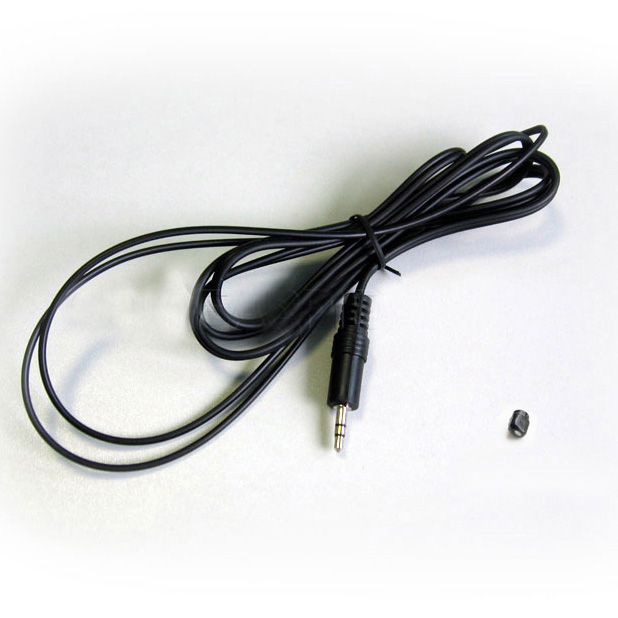This photograph depicts a black 3.5mm auxiliary cord, which appears coiled and secured with a black zip tie, laying against a white background. The coiled cord has a flexible black rubber or plastic exterior and is attached to a silver 3.5mm plug with two black rings near the end. To the right of the plug, there's an indistinct small black plastic element, whose function isn't entirely clear from the image. Notably, only one end of the cord, featuring the 3.5mm jack, is visible in this photograph, and the other end remains out of view.